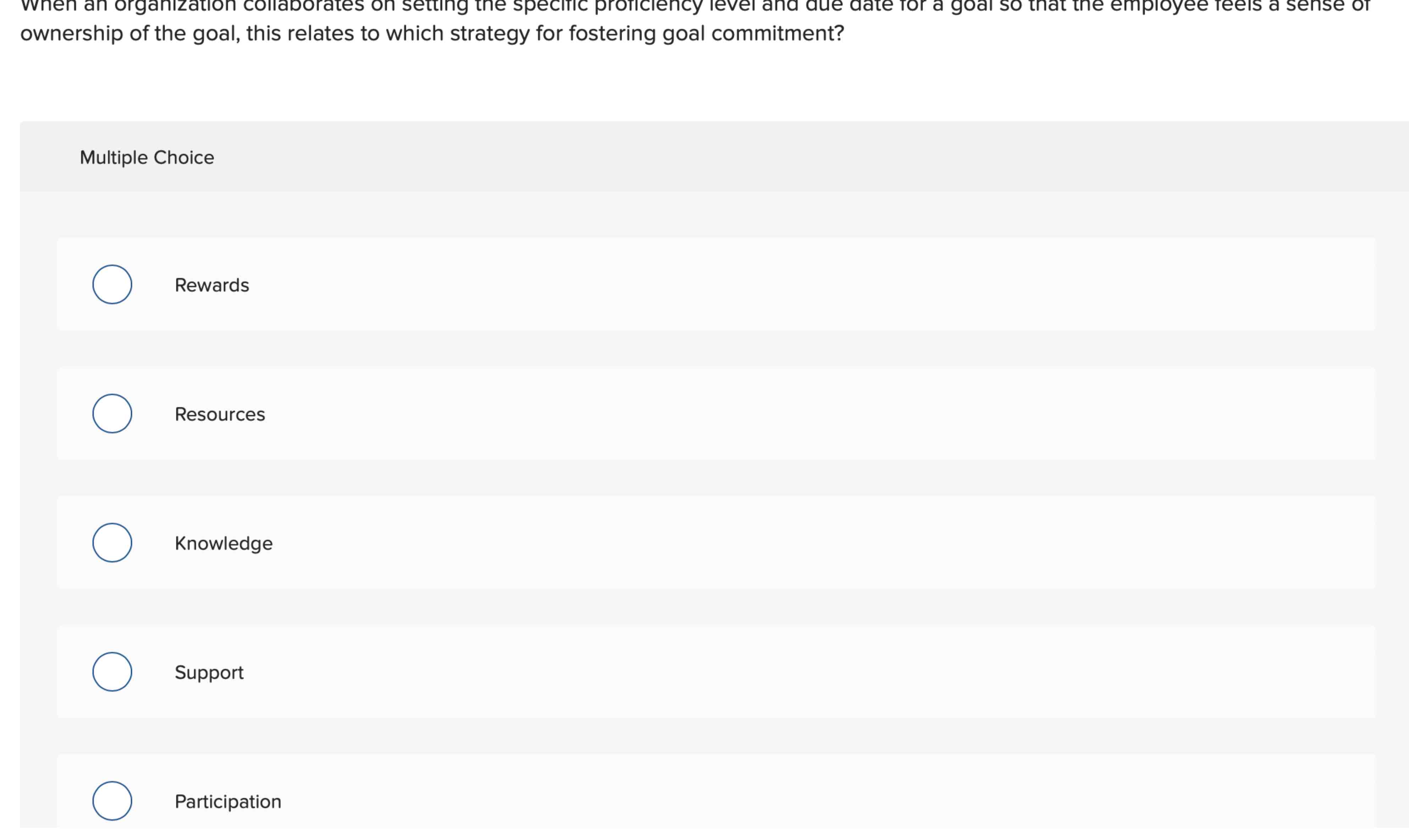This image is a screenshot from what appears to be a computer-based exam or quiz. The lower part of the image features a grey box headed with the words "Multiple Choice" on the left. Above this grey box, the image displays two lines of text ending in a question, indicating this is one of the questions from the exam. Unfortunately, the top of the letters in this text is cut off, which makes it partially obscured. The visible portion of the question reads: "When an organisation collaborates on setting the specific proficiency level and due date for a goal, so that the employee feels a sense of ownership of the goal, this relates to which strategy for fostering goal commitment."

Below this question, the grey box is divided into five segments, each containing a possible answer. Each answer is presented on a white banner set against a lighter grey background. To the left of each banner is a selectable circle. The answer choices are as follows:

1. Rewards
2. Resources
3. Knowledge
4. Support
5. Participation

These options are designed to be selected by clicking the circle next to the corresponding word. It is not clear whether there are any additional options beyond these five, as the visible portion of the image only shows these.